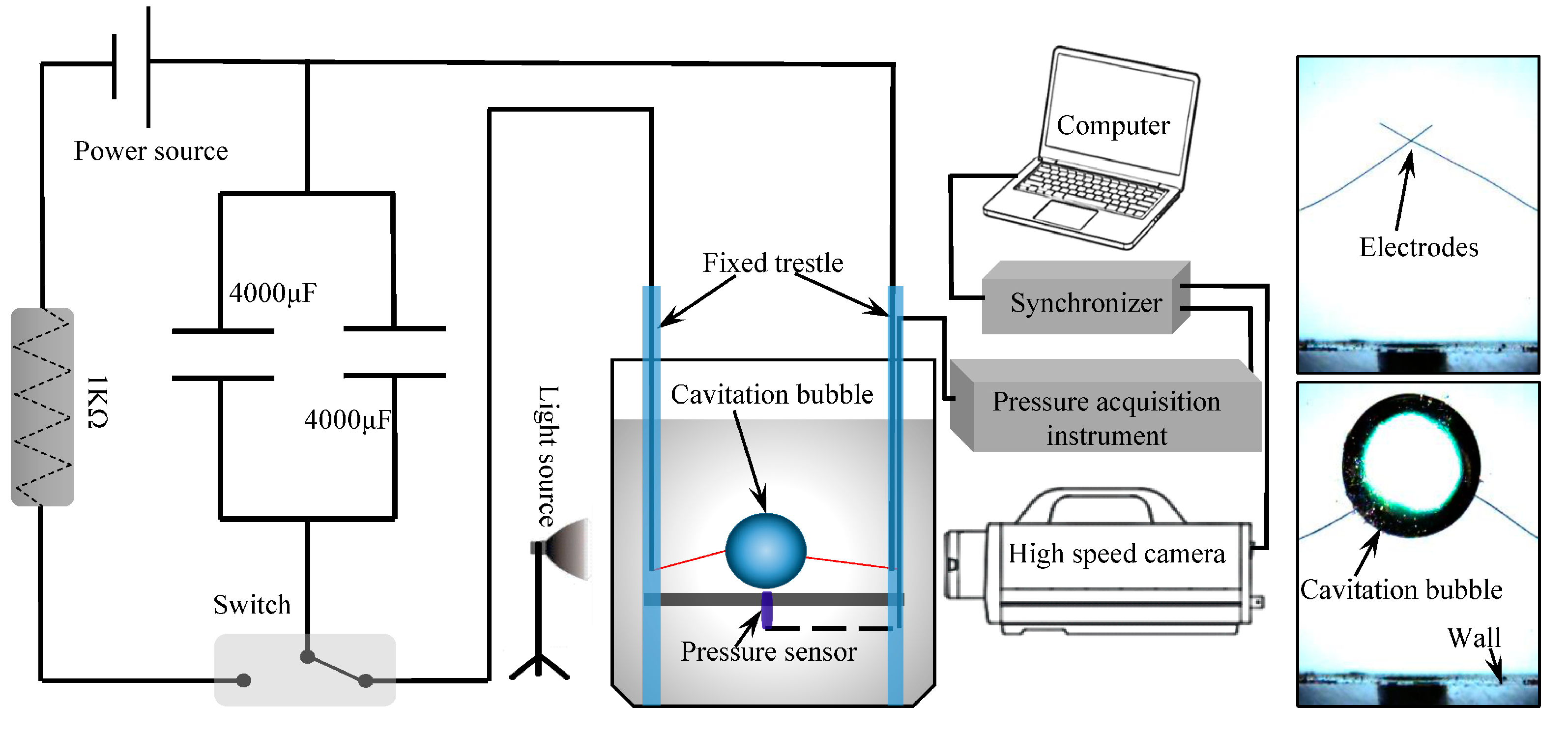This image is a detailed flowchart diagram illustrating the process of electricity traveling through various components to power items. A thin black line outlines a square shape, connecting a multitude of elements in a sequence. Key components include a power source, a synchronizer, and numerous labeled items such as a cavitation bubble, high-speed camera, and a pressure acquisition instrument housed in a gray 3D box. Symbols like the omega sign and numerical values such as 4000UF are present, alongside images of a laptop computer and electrodes. Multiple arrows direct the flow to indicated components. The diagram, though complex, seems to emphasize the process involving power sources, synchronization, and capturing data or images with specialized equipment.